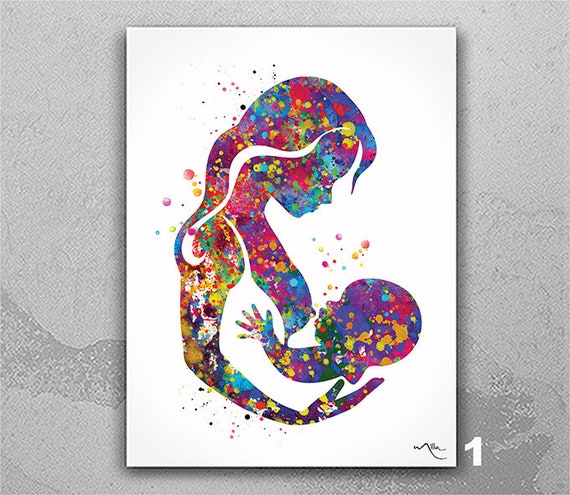In this detailed painting, which rests on a dark and light grey marble-textured surface, we see a white poster board featuring a vibrant and captivating mosaic artwork. The painting portrays a side-view silhouette of a woman with long hair, possibly wearing a sleeveless slip, cradling a baby in her arms in an intimate breastfeeding moment. This poignant scene is depicted entirely through an intricate arrangement of colored dots without the use of lines, showcasing colors such as yellow, blue, red, green, purple, pink, and white. These dots are randomly placed, yet they come together to form a cohesive image. At the bottom right corner of the poster board, there is a light-colored number "1" and a barely discernible black squiggle that appears to be the artist's signature.